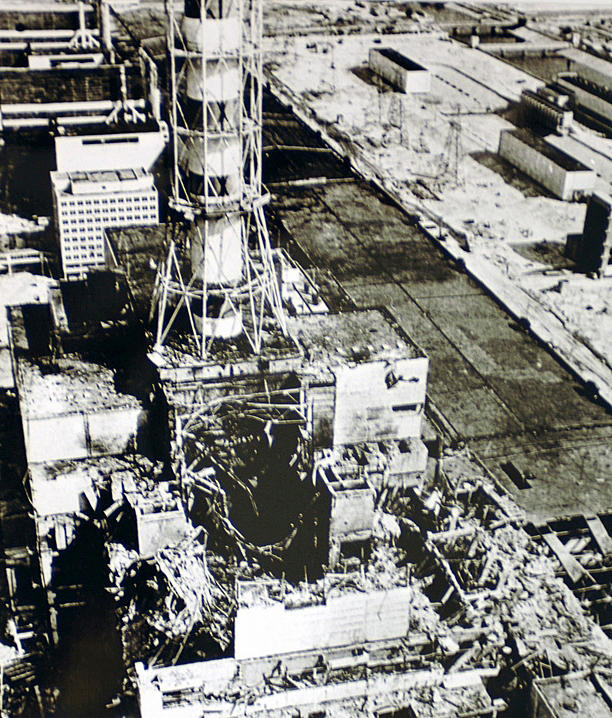The image is a grainy, black-and-white aerial photograph depicting the aftermath of a catastrophic event, likely at Chernobyl. The view is from above, possibly taken from an airplane or helicopter, capturing a scene of widespread destruction. The most prominent feature in the image is a large building with a gaping hole in its roof, surrounded by twisted metal, debris, and rubble, indicative of a powerful explosion, possibly from the reactor meltdown.

To the right of the ruined structure, smaller buildings and trailers are visible, while the left side features an industrial area with taller buildings and a prominent spiral tower. The destruction is concentrated in the lower part of the image, where debris and metal fragments are scattered amidst what appears to be dusty, gravel-strewn terrain. The entire scene is monochromatic, enhancing the stark and somber atmosphere of the devastation.